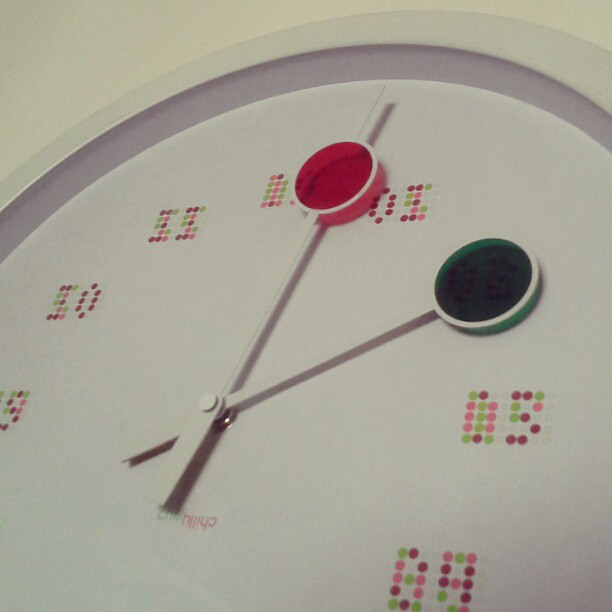The image features an ultra-modern clock in an extreme close-up shot, capturing only its upper half. The clock, circular in shape, boasts a minimalist and monochromatic design with a white background, white rim, and white face. The numbers on the clock face are distinctly pixelated and displayed in a digital, binary style, featuring red digits such as "01," "02," "03," and "04." While the lower numbers are not visible, the upper numbers from "09" to "12" can be seen clearly. The clock hands are strikingly unique, resembling lollipops with a red minute hand and a green hour hand, indicating the time is approximately two o'clock.